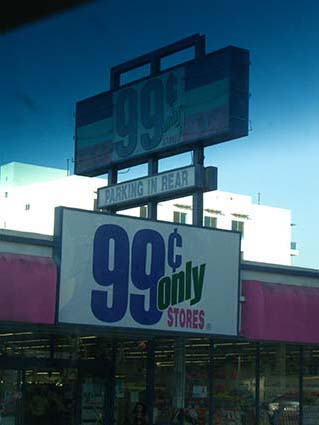A vibrant storefront is depicted, showcasing the signage of a "99 Cents Only Store." The prominent sign above the entrance features multi-colored text with the number "99" in blue, the word "only" in black, and "stores" in a shade that appears red or pink, though the exact colors are hard to distinguish due to dim lighting. Above this main sign, an elevated sign reads "Parking in Rear" with additional phrasing related to the 99-cent theme. The storefront's upper facade is painted in red or pink, while beneath it, large glass windows provide a glimpse into the store's interior, though specific details are obscured. In the background, a larger, white building looms above the store, adding depth to the scene.